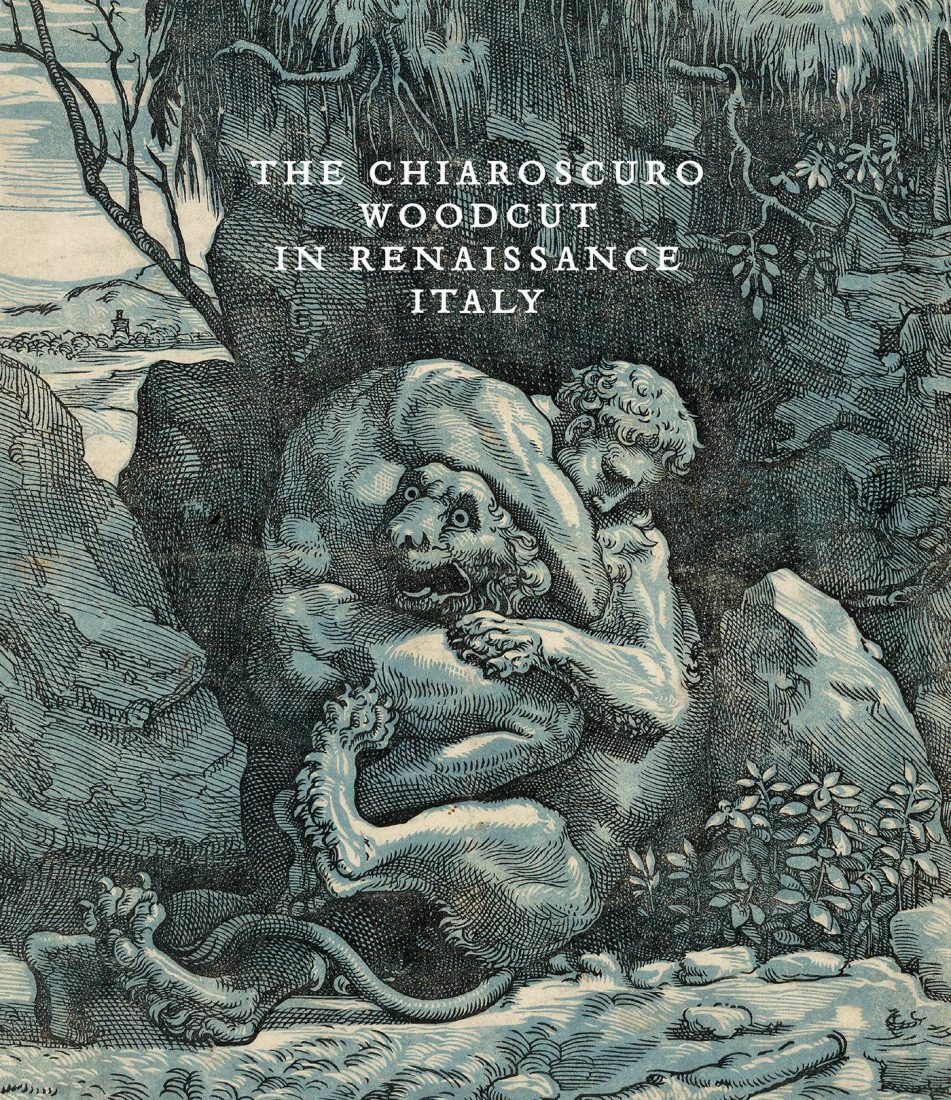This image, appearing as the front cover of a children's illustrated book titled "The Chiaroscuro Woodcut in Renaissance Italy," depicts a detailed black, beige, and white woodcut or engraving. At the center, a muscular, unclothed man, resembling a statue from the 15th century, is fiercely bent over, wrestling a lion-like creature. The man, looking determined, has the lion in a headlock, with his knee pressing into its chest. The lion, with a humanoid yet leonine face, appears frightened, its eyes wide and mouth open in distress. Surrounding them is a rugged landscape with rocks, pebbles, vegetation, and the roots of tall trees and a cliff. In the top left quarter of the image, blurred in the distance, there is a small house nestled in a valley. The entire scene is rendered in a style reminiscent of newspaper illustrations, combining elements of classical and Renaissance art with an intricate depiction of nature and struggle.